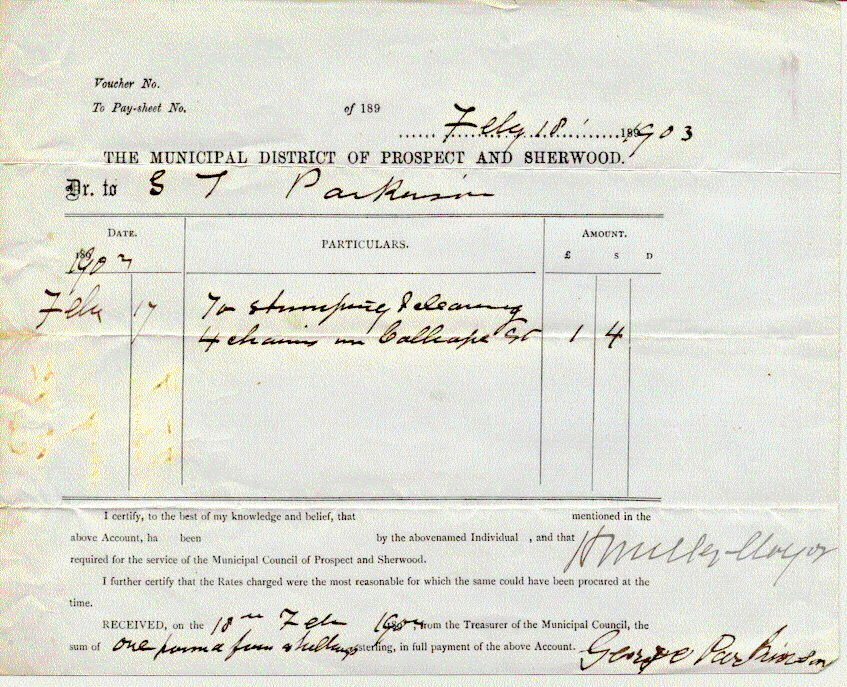This image depicts a digital screenshot of an aging, worn voucher that appears to be an official document from the Municipal District of Prospect and Sherwood, dated February 18, 1903. The voucher, showing significant signs of age with stains and a prominent crease indicating it was once folded neatly in half, is difficult to decipher due to its faded state. The text includes several legible sections: at the top, it reads "Municipal District of Prospect and Sherwood," followed by the payee line, on which "ST Parkinson" is inscribed. The voucher references a payment sheet number and contains a certification statement verifying that the account was serviced by the named individual for municipal purposes. The document is signed and further certifies that the rates charged were the most reasonable at the time. A final note mentions a receipt by the Treasurer of the Municipal Court, but the specific details remain mostly illegible. The voucher's historical and geographical context suggests it originates from the UK.